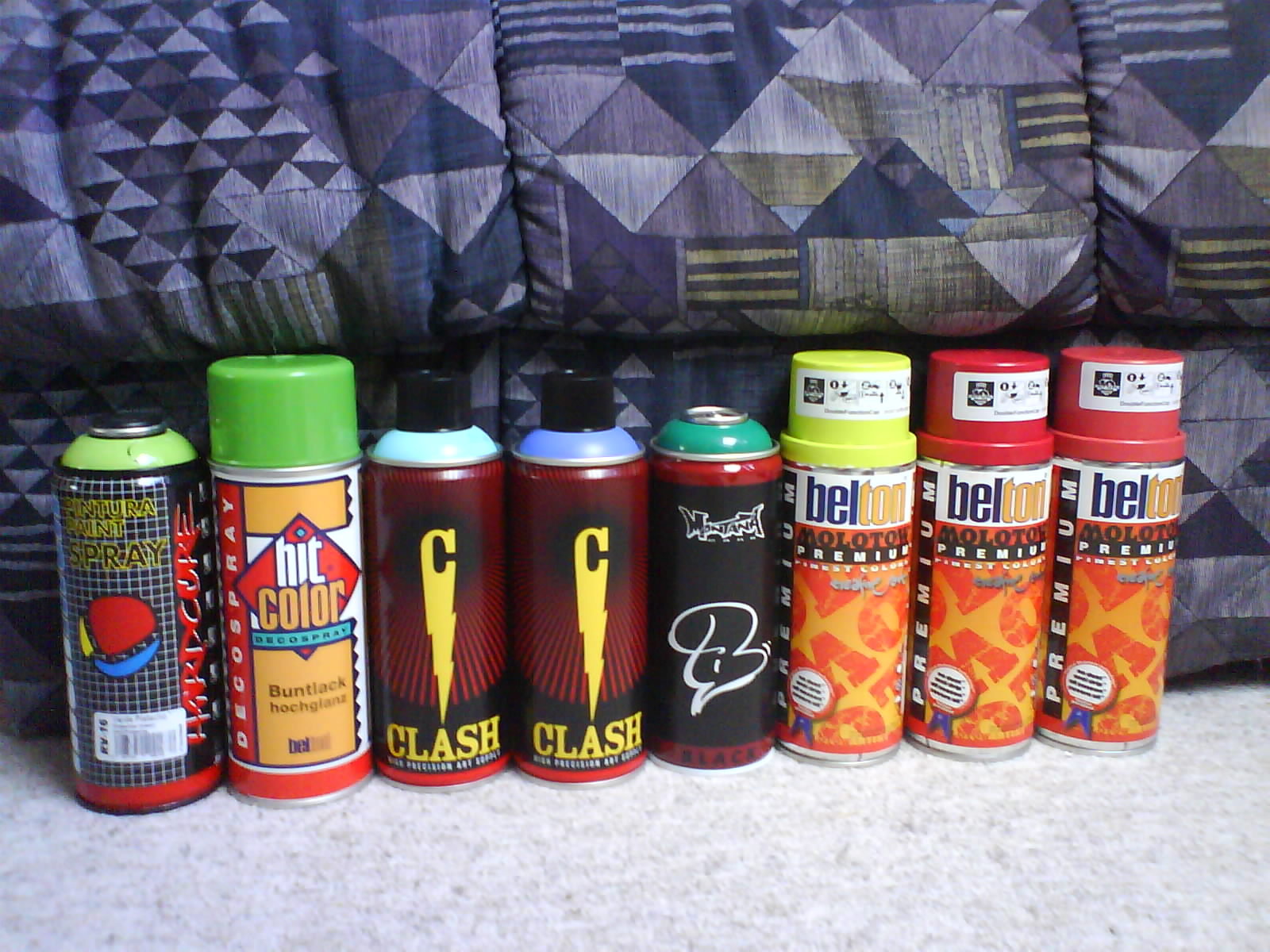The photograph showcases eight spray paint cans, arranged side by side on a white vinyl floor. Behind the cans lies a quilted material resembling a sleeping bag, decorated in geometric patterns with shades of black, grey, silver, and dark olive green. The eight cans vary in color, brand, and design. On the far right, there are three identical Belton Molotow Premium cans, each with red, fluorescent yellow, and a distinctive green cap. To their left, a black can marked with a stylized letter 'B' sits without a cap and features a number three along with "Montana" written in white. Two identical Clash-branded cans with black caps and a yellow 'C' with a lightning bolt design follow next. The second can from the left, labeled "Hit Color", sports a red design with yellow accents and a bright green cap while the leftmost can displays a multi-colored design with red, blue, and yellow hues, featuring the text "Ventura Paint Spray" and "Hardcore" alongside a white sticker with black text.